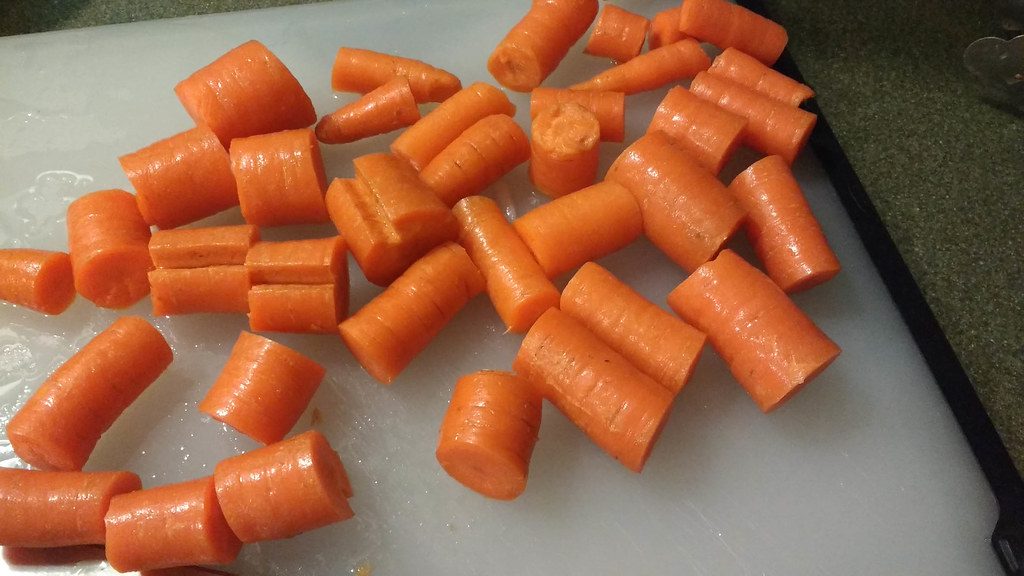In this detailed close-up photograph, 36 pieces of freshly washed, unpeeled carrots are arrayed on a wet, white plastic cutting board with black edges. The carrots, varying in size, are chopped into a mix of round cylindrical chunks and longer lengthwise pieces, with some segments split and cracked open, revealing their natural interior texture. The cutting board, streaked with shadows giving it a slightly grayish tint in places, is set on a greenish-gray granite countertop adorned with white and black speckles. The glistening carrots reflect light, underscoring their shiny, moist appearance. In the background, the right-hand side of the image hints at kitchen tools, possibly including a knife, suggesting recent chopping activity.